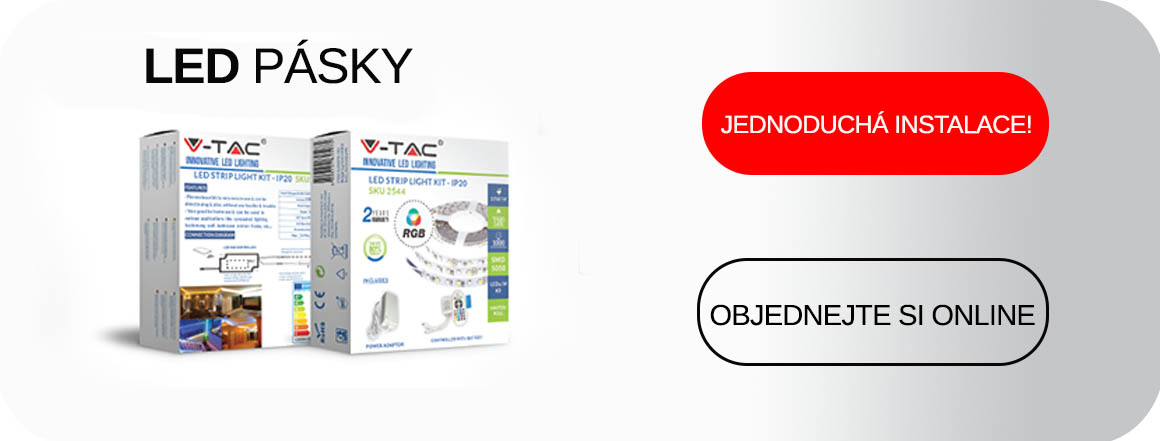The image appears to be an advertisement for LED strip lights, prominently featuring the product inside two boxes against a gradient gray background that transitions from lighter on the left to darker on the right. In the upper left-hand corner, "LED PASKY" is written in bold, black font, with "LED" emphasized. The boxes are labeled "V-TAC" in the upper right-hand corner and are white with blue text detailing the product. The front and back views of the packaging are displayed, filled with busy text and descriptions, likely in another language, indicating its features and usage. To the right of the boxes, there is a red, clickable button with white text that reads "JETNODUCA INSTALANCE!" Below it, there is a clear, pill-shaped button outlined in black with black text that reads "OBJENDENEDCY ONLINE." The image overall looks visually comprehensive, aiming to convey detailed information about the LED strip lights and how they can be installed or used.